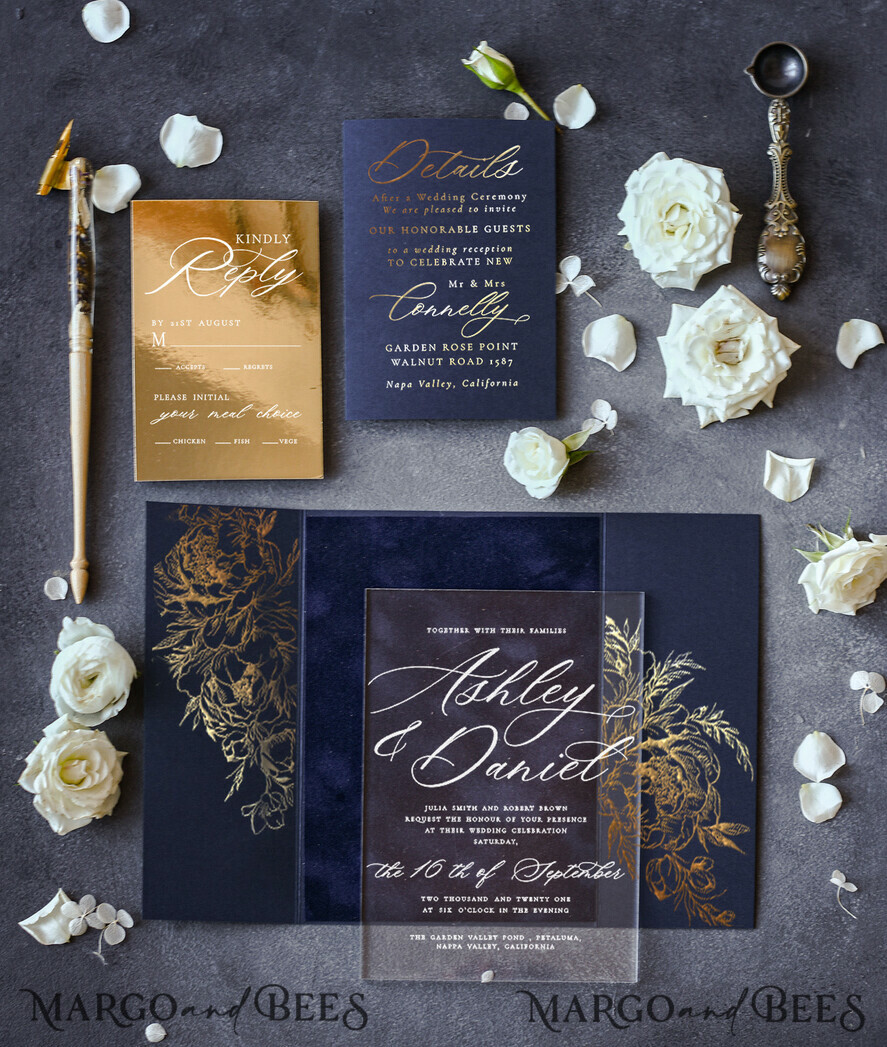The image is a meticulously arranged collage-style display designed for a wedding, specifically for Ashley and David. The background transitions from light gray in the center to dark gray at the bottom, adding an elegant gradient effect. Prominently featured are several white roses and scattered petals. The bottom left and right of the image both display the text "Margot and Bees."

Among the items included are three ornate pamphlets: a golden one, a blue one with gold cursive writing, and another that appears to be an RSVP card. Additionally, there is a card detailing the location of the wedding. An antique silver spoon is positioned toward the top right of the display. There is also an ivory-colored object, possibly a crochet hook or an embossing tool, situated on the left-hand side.

At the center of the collage, a rectangular piece of glass elegantly displays the engraved wedding invitation. The overall aesthetic combines a classic floral theme with vintage and intricate elements, exemplified by the ornate envelopes and detailed pamphlets, creating a beautiful and sophisticated visual for a wedding invitation.